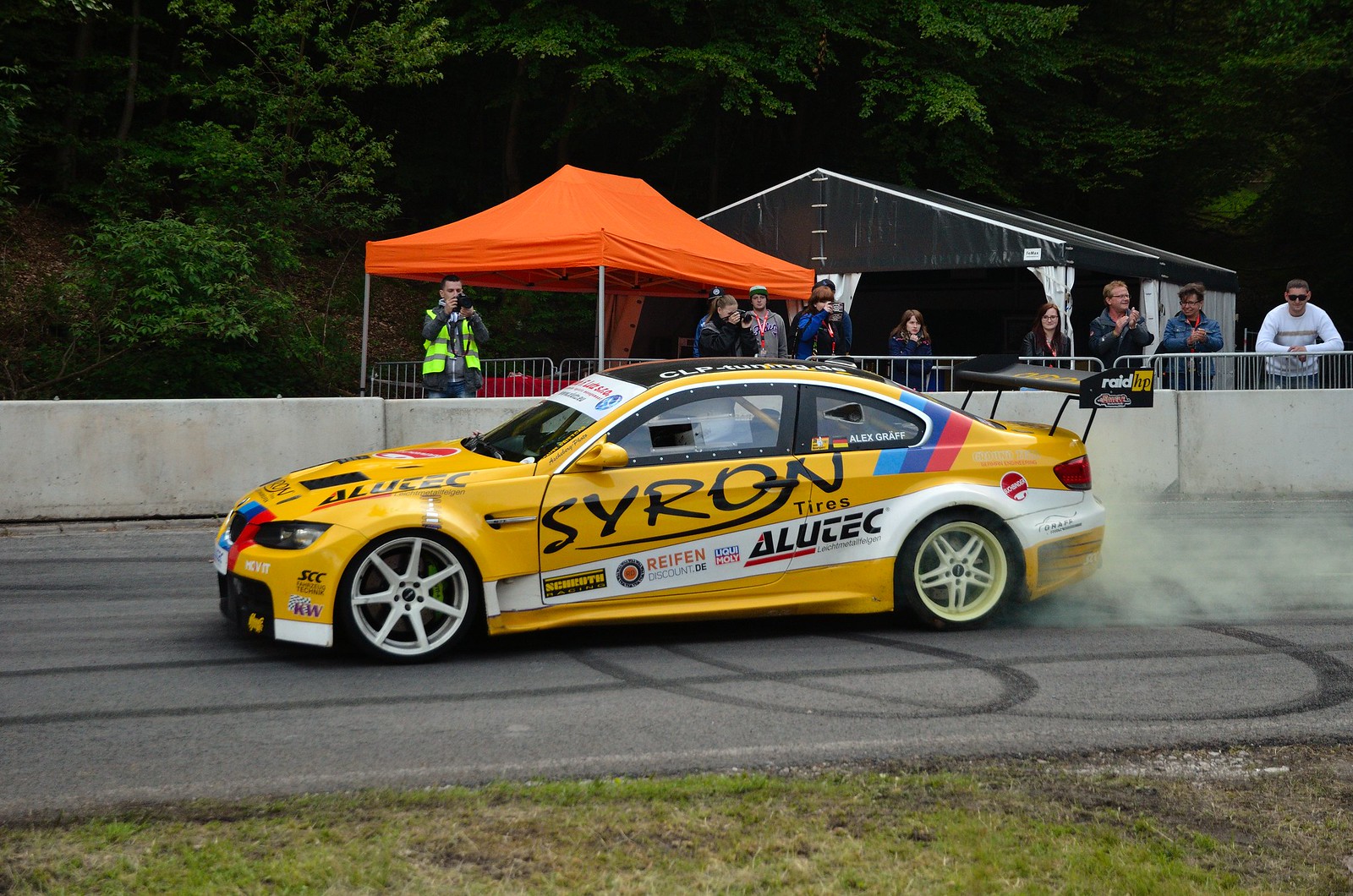The image showcases a dynamic and action-packed moment at an outdoor motorsport event. At the center of the scene is a yellow sedan, identified as a rally type car, caught in the midst of a dramatic drift on a black tarmac track. Smoke billows from beneath the car, suggesting it is burning rubber as it powers through the turn. The car, possibly a BMW, features notable details such as large white rims, a black metal spoiler, and prominent black lettering on the door panel reading "S-Y-R-O-N." Advertising text adorns various parts of the bodywork.

In the background, a small concrete barrier wall and metal fencing frame the scene, providing a clear boundary for safety. Spectators, wearing colorful clothing, including lime green safety jackets, are positioned behind the fencing and appear fully engaged, some taking photographs and others simply observing the race. The vibrant colors of their attire contrast with the muted tones of the safety barriers. Additional elements include an orange awning on thin aluminum poles and a black awning with white drapes, both providing shelter for more onlookers. The foreground features green grass with patches of black dirt, adding to the authentic, rugged atmosphere of the motorsport event.